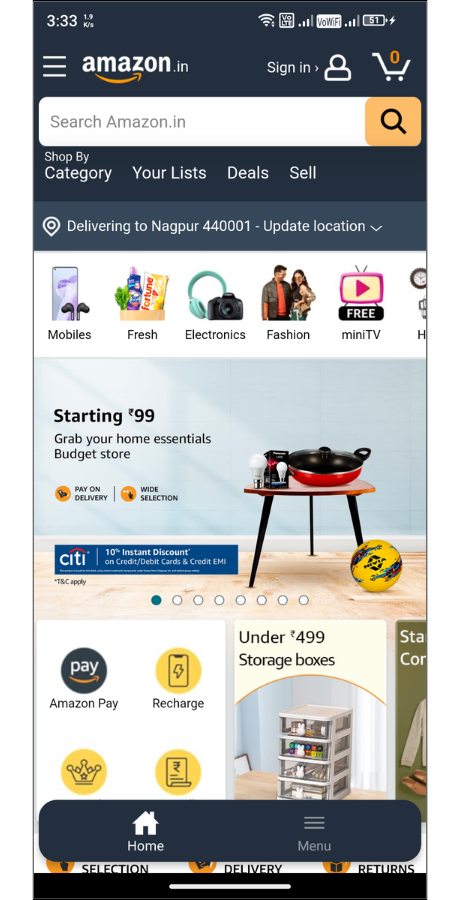A detailed caption describing the image of Amazon.in being viewed on a smartphone:

The image displays the Amazon.in homepage as seen on a smartphone at 3:33 PM. The device shows a full Wi-Fi signal, VOLTE indicator, and a battery level of 51%. At the top of the screen, there is a hamburger menu icon, followed by the Amazon logo, a sign-in icon resembling a person, and a shopping cart icon indicating zero items. Below this, a search bar with the placeholder text "Search Amazon.in" is present, accompanied by an orange search button with a magnifying glass icon.

Just beneath the search bar, there are navigation tabs labeled "Shop by Category," "Your List," "Deals," and "Sell." A lighter field follows, showing the delivery location as "Delivering to Nagpur 440001" with an option to update the location. The main content area features thumbnails of various categories including a phone with speakers, headphones labeled as "Mobiles, Food & Fresh," a camera under "Electronics," two people representing "Fashion," and a TV icon for "Amazon Mini TV." Some text and images are slightly cut off on the right.

Further down, there's an image of cookware and light bulbs on a stool with text that reads "Starting at ₹99, grab your home essentials. Budget store, pan delivery, wide selection, city card option." Underneath, there are eight more options available for browsing. At the bottom section of the screen, there are logos for Amazon Pay, and an advertisement for storage boxes priced at ₹499. The bottom navigation bar includes a home button and a menu button.